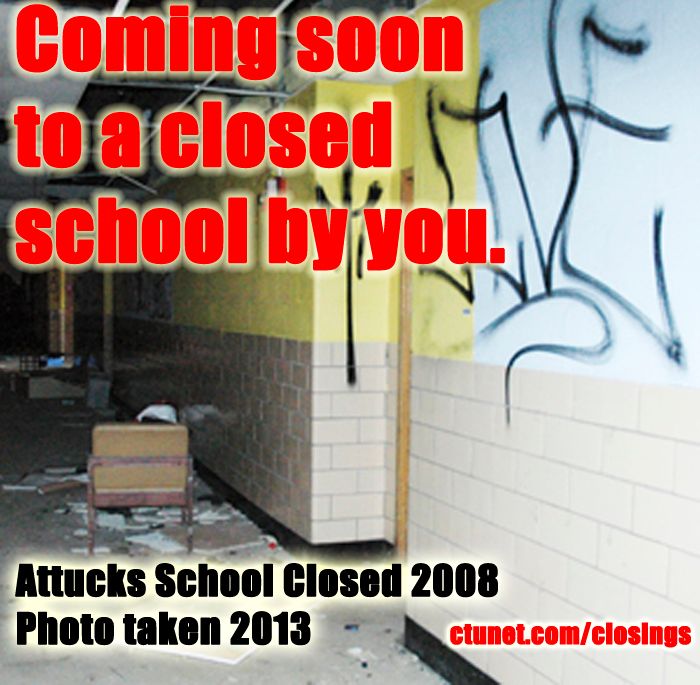The image is a graphically enhanced photograph showcasing a vibrant, urban scene. The focal point is a wall divided into two color schemes: a light blue section on the right transitioning into a yellow section on the left. This division is punctuated by a doorway in the middle, featuring a dark brown wooden door. Below these colorful sections is a tan, unpainted brick wall, which also bears graffiti that stretches across both the blue and yellow portions.

At the base of the brick wall is a black strip along the floor, providing a stark contrast to the colors above. A circular watermark with intricate swirls and the text "photobucket" is visible, marking the image's source.

Overlaying the walls and graffiti are various text elements in bold, eye-catching colors. At the top, red text with a white accent reads "Coming Soon" on the first line, followed by "A Closed" on the second line, and "School Near You" on the third line. Below this text, a slightly opaque rectangle reveals the image of an orange and red chair in the background.

In black text with an exclamation mark, the phrase "Protect more of your memories for less!" is prominently displayed. On the left-hand side, black text on a yellow background announces, "Attacks School Closed 2008" and further details with "Photo taken 2013" on the next line. The far right of the image features red text with a white shadow, displaying the web address "c-t-u-n-e-t ctenet.com/closings".

This detailed caption thoroughly describes the elements within the image, highlighting both its artistic and informational aspects.